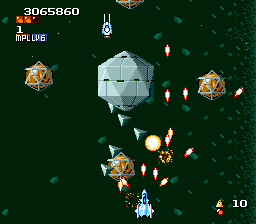The image appears to be a screenshot from a retro, Atari-style video game set in space with a pixelated aesthetic. The backdrop is a green field punctuated with various symbols and particles. The most prominent feature, centrally located, is a large gray-silver spaceship with an octagonal, almost diamond-shaped design. Surrounding it are mini-spaceships shaped like jeweled diamonds, also engaged in combat, firing red and yellow bullets that leave green trails. 

In the top left corner, the score is displayed as "3065860" in white text. Directly below this, there are three amber square boxes with two illuminated, alongside a numerical "1" beneath them. Additionally, there is an inscription "MPL" on a brown background underneath the "1," with "LV6" next to it on a blue background. 

In the bottom right corner, a golden triangle with a red circle appears above the number "10" in white font. At the very bottom, a centrally positioned fighter jet, white with blue trim, points upward, seemingly shooting at the central octagonal object. The left side of the scene also features two brownish trees and another black tree with a red border.